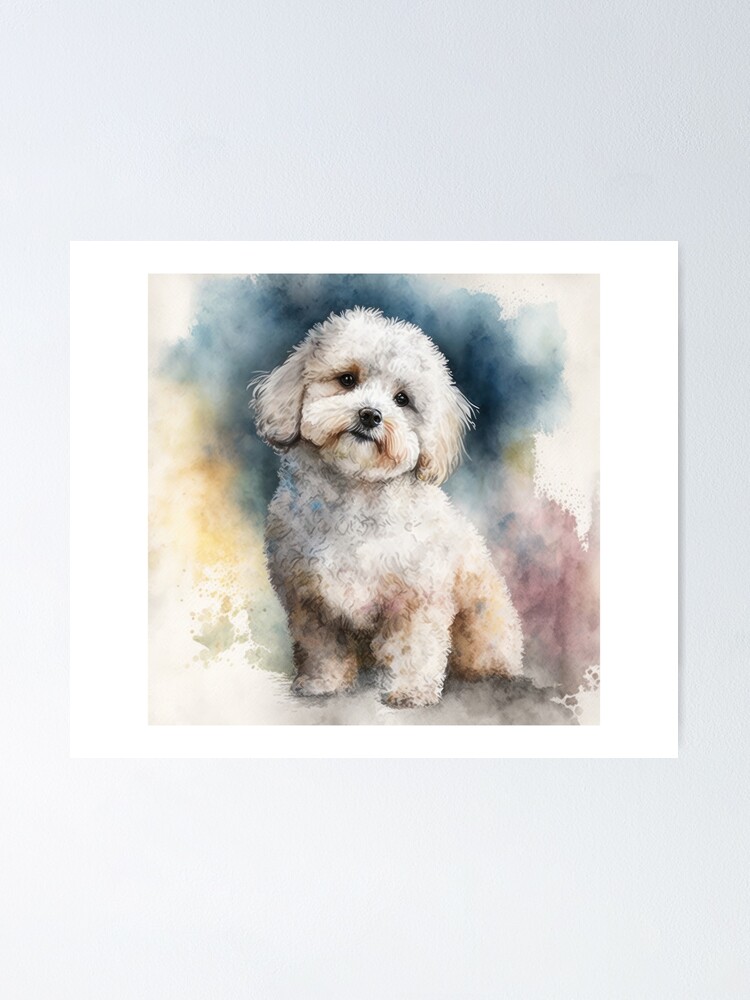The image is a watercolor painting depicting a small, white, fluffy dog with dark eyes and a dark nose, sitting and looking at the viewer. The dog has short, hanging ears and subtle brown shading around its jowls and the inside of its front and back legs. The background features clouds of various colors: a dark blue cloud at the top surrounding the dog's head that fades out towards the edges, yellow on the sides, pink at the bottom, with additional accents of grey and red. This detailed aura creates a vibrant and dynamic setting for the dog. The painting itself is a slightly rectangular square mounted on a white mat, which is then framed by a taller grey background. The overall framing and colorful surroundings highlight the dog, making this a captivating piece of artwork, effectively combining aesthetic appeal with the charm of a beloved pet.